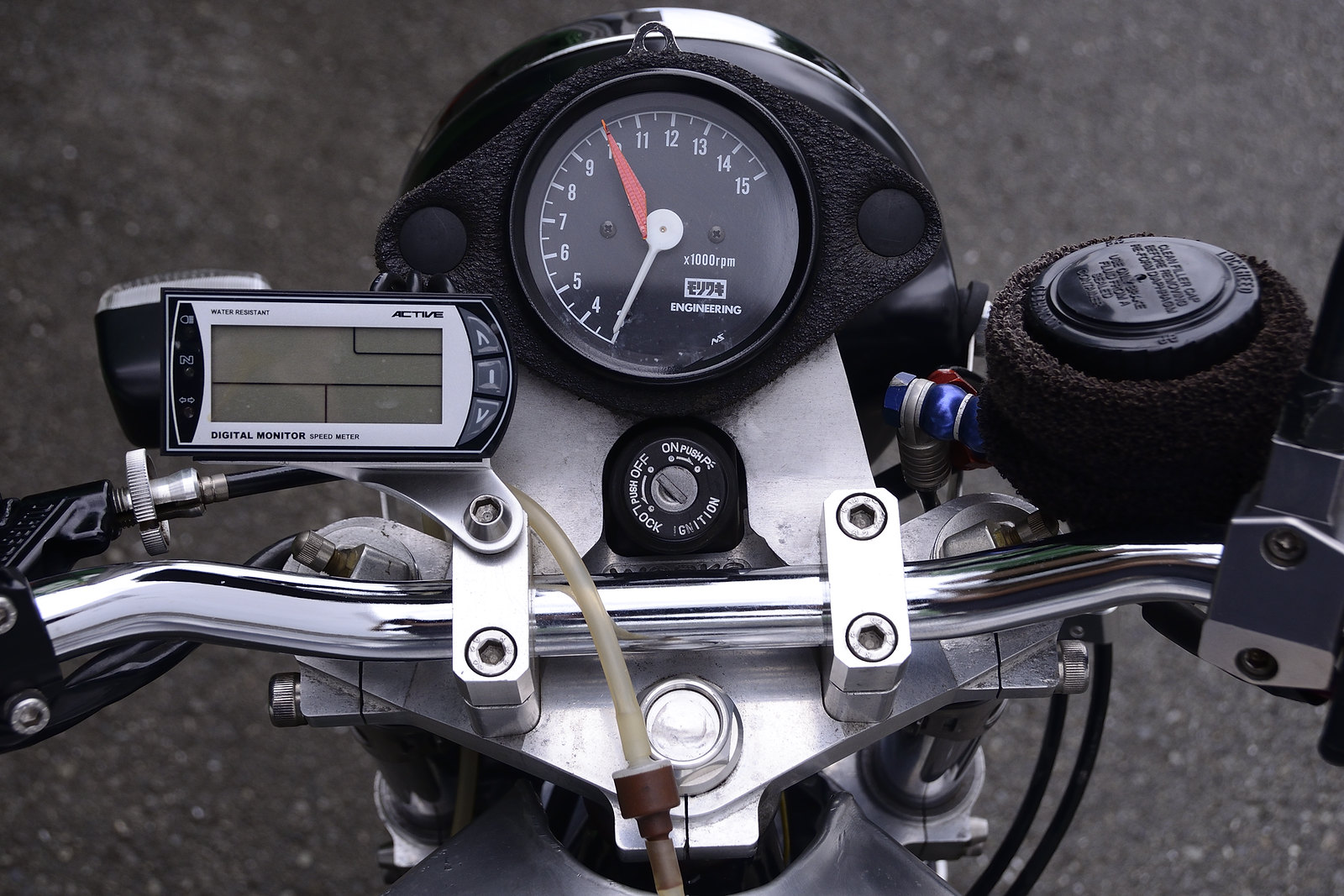This close-up photograph showcases the intricate arrangement of devices on the handlebars of a motorcycle. Dominating the frame is a pristine chrome bar, parallel to the bottom, which flares slightly downward along each side. This bar seamlessly connects to an angular, matte metallic surface. 

At the core of this setup is a prominent silver keyhole, outlined in black. Encircling the keyhole are white text labels in a clockwise direction, starting from the 12 o'clock position: "ON," followed by "PUSH," "P," "IGNITION," "LOCK," "PUSH," and "OFF." An arrow indicates the transition from "OFF" to "LOCK" and then to "P."

Above the keyhole is a round gauge with a black background and a sleek, shiny black rim. The meter spans an arc from around seven o'clock, starting at zero, up to about two o'clock, peaking at fifteen. A red needle points toward ten while a silver needle rests at zero. Adjacent text reads "× 1000 RPM," accompanied by Japanese characters in black on a white strip, and the word "ENGINEERING" in white text below.

To the left, there is a digital screen with a silver outline, adorned with black buttons. The screen's labels include "WATER RESISTANT" at the top left, "ACTIVE" at the top right, and "DIGITAL MONITOR SPEED METER" at the bottom left.

On the right side of this setup, there is a black button or dial with black text. The text inscribed reads, "Clean filler cap before removing reformed diaphragm," instructing to "Use only brake fluid from a sealed container," alongside the brand name "Lockheed" on either side.

This meticulous assembly of devices highlights the complex functionality and engineering precision characteristic of modern motorcycles.